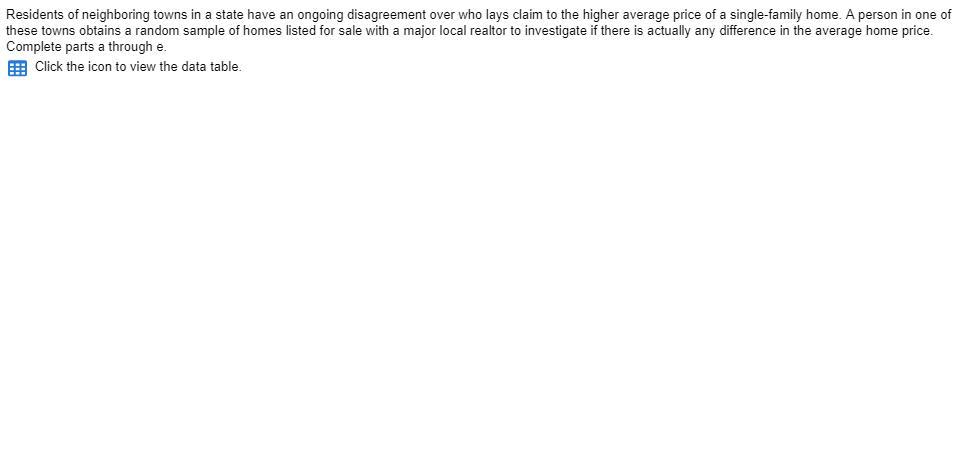The image features a predominantly white background with black text detailing a dispute among residents of neighboring towns in Texas regarding which town boasts a higher average price for single-family homes. To investigate this claim, a resident from one of the towns takes a random sample of homes listed for sale through a major realtor. The image includes a blue calendar icon with an adjacent message in black text instructing viewers to click the icon to view the table. The remainder of the screen is largely blank, providing ample whitespace. The creator expressed a hope for financial rewards from their efforts to be approved so they could access funds for groceries, indicating a delay in the approval of their recent activities, including watch and typing tasks.